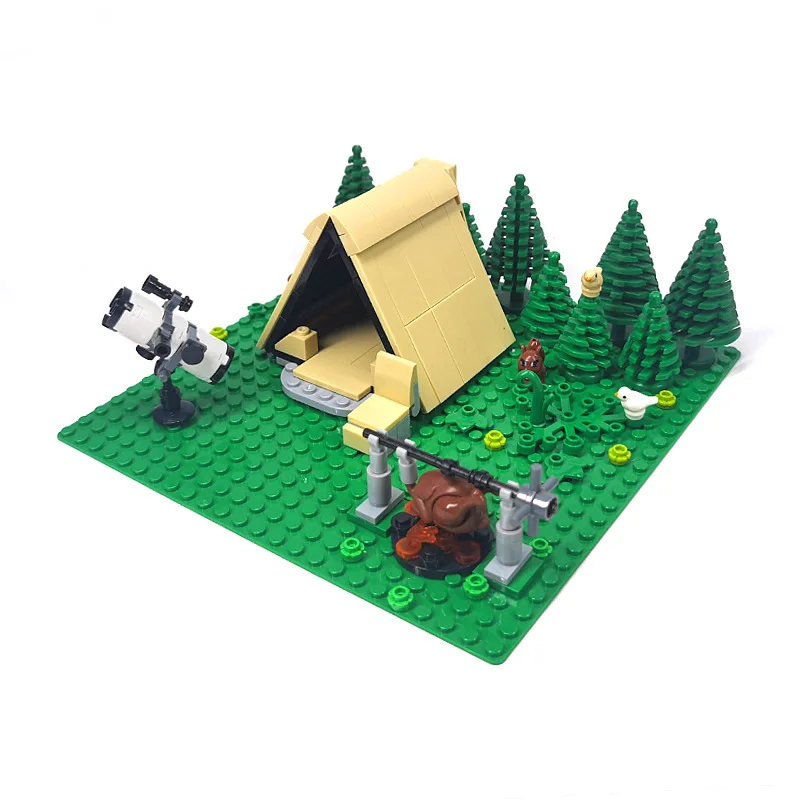The image showcases an intricate Lego camping scene set on a green Lego board resembling grass. Dominating the background are seven Lego trees designed to look like conifer or pine trees, one of which has a yellow bird perched on top. Beneath this tree, there is a brown Lego squirrel next to a white Lego bird. In the foreground, a tan Lego tent stands prominently with a light brown chair positioned just outside it. Close to the tent, a white and black Lego telescope is mounted on a stand, seemingly pointed towards the sky. Directly in front of the tent, a silver-gray and black Lego spit roast features a brown turkey (or possibly a chicken) cooking over a Lego fire. Altogether, the scene artistically recreates a tranquil camping environment, complete with detailed wildlife and camping gear elements.